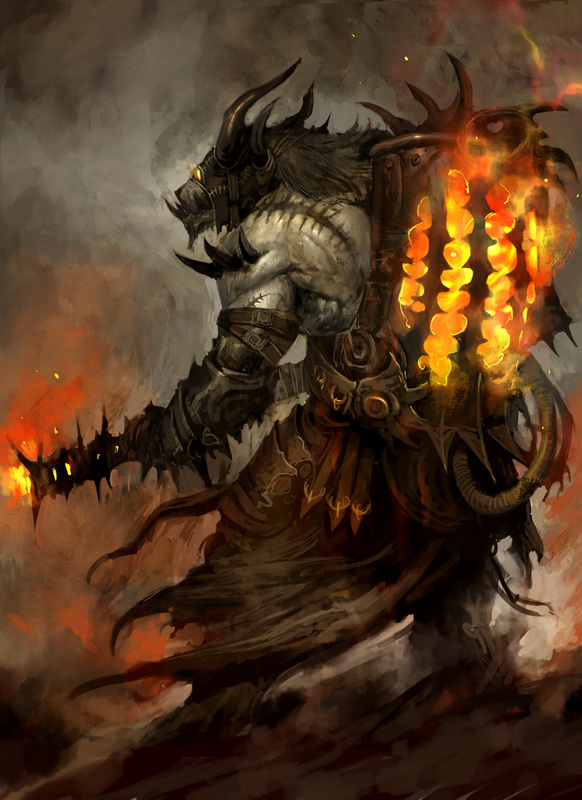The image depicts a detailed fantasy scene likely inspired by a medieval-oriented video game. The central figure is a monstrous creature with a head resembling a horned wolf, featuring fangs and glowing yellow eyes. It is arrayed in a mix of silvery armor on its chest and upper arms, and tattered garments that include a kilt-like piece adorned with metal facets, suggesting a blend of both uniform and rugged attire.

This formidable beast wields a flamethrower, with flames vividly active in a brass cage-like backpack, from which they travel down to the instrument it holds, projecting fire out of its tip. The creature's overall appearance is characterized by dark colors, with spikes jutting out from its form and additional horns emerging from its left shoulder. It stands against a chaotic, smoke-filled backdrop, where shades of gray, black, orange, and brown intermix in a fiery swirl, contributing to the image's intense and ominous atmosphere. The creature is intent and focused, looking and pointing towards the left, as floating debris or embers drift in that direction. This intricately painted scene captures a moment of fierce confrontation within a foggy, mist-laden background, bringing the fantasy world vividly to life.